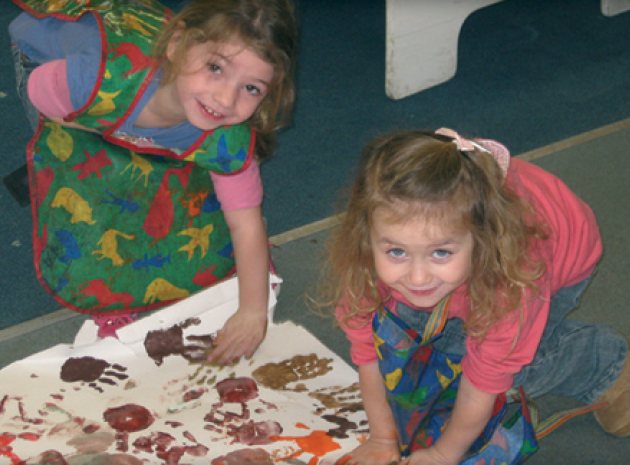This photograph captures a delightful moment of two young girls engaged in creating a handprint collage. Set against a dark blue wall, the room features a lighter green floor with some white patterns visible. The focal point is the large piece of white poster paper on the floor in front of them, already adorned with various colorful handprints. Both girls are on the floor, posing for the camera with joyful expressions. 

The girl on the left, slightly leaning over with her left hand on the paper, has brown eyes and dirty blonde hair. She is wearing a pink shirt and a painter's smock decorated with fish. The girl on the right, also with dirty blonde hair but with blue eyes, is in a similar pink shirt paired with blue jeans. She is kneeling with both hands pressing into the paper. 

Both girls are donned in typical preschool-style plastic aprons to protect their clothes from paint. They seem to be having a wonderful time, fully immersed in their creative activity.